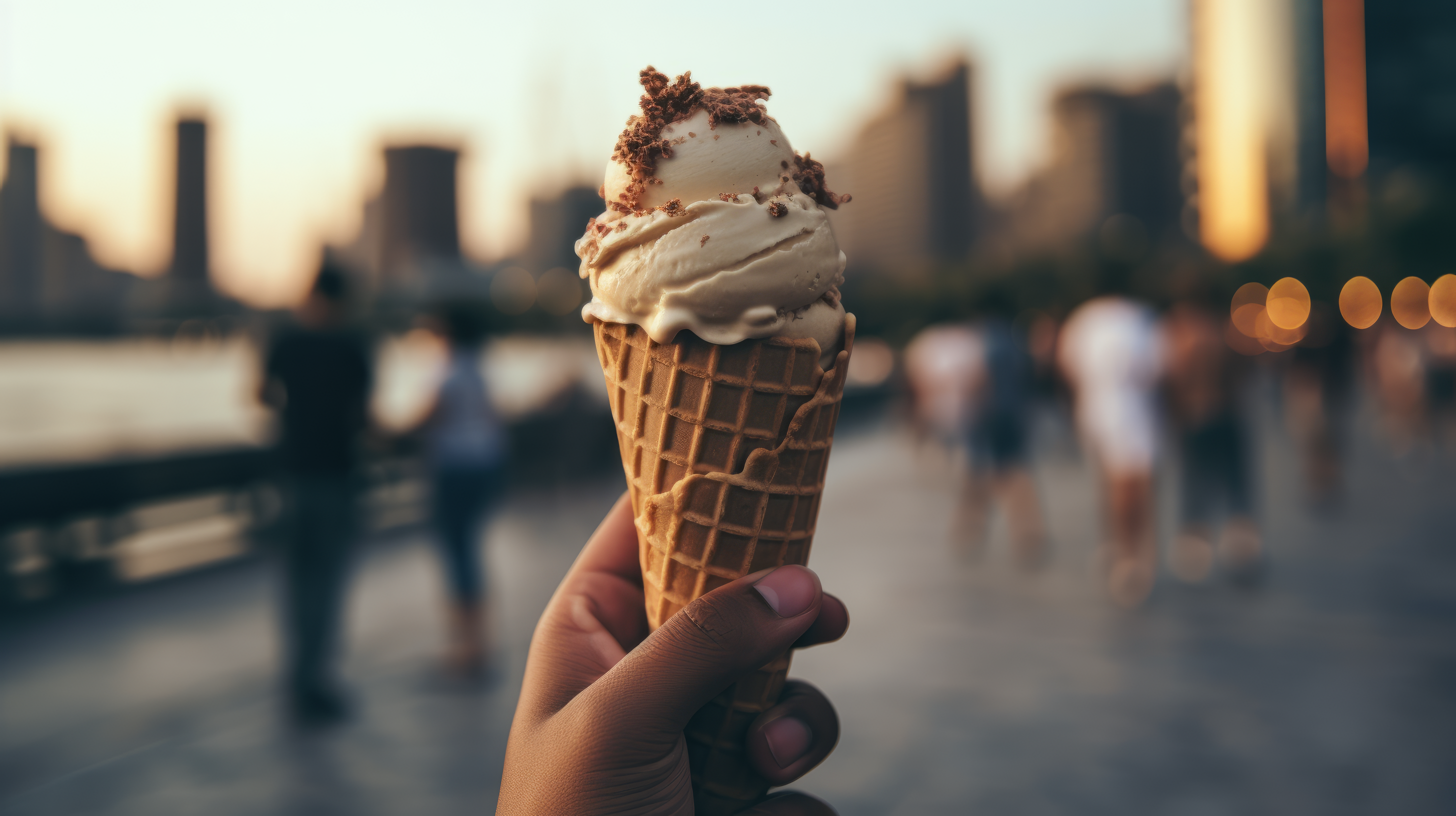In this detailed photograph, a hand, likely belonging to an African American male, is prominently holding a vanilla ice cream in a waffle cone. The ice cream is topped with what appears to be brown crumbles, which could be nuts or cookie crumble. The foreground is in sharp focus, while the background features a blurred cityscape at sunset, with high-rise buildings silhouetted against a warm yellow sky. People can be seen in the softened backdrop, leisurely hanging out by a body of water, possibly a lake or stream, adding to the urban yet serene atmosphere. The overall ambiance suggests a calm, evening scene in the city.